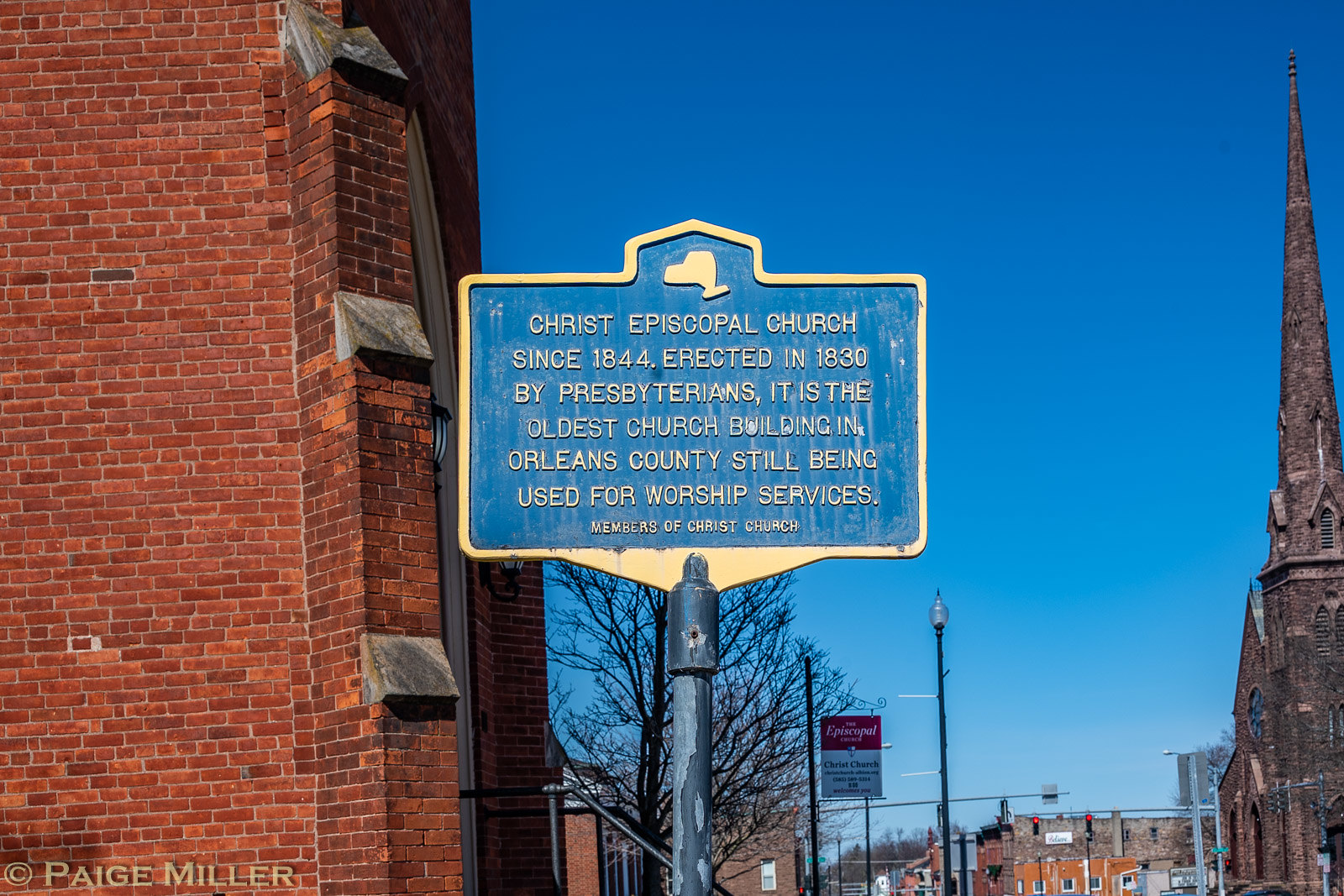The photograph captures a detailed scene featuring a historical sign positioned on a sidewalk in front of a large, brick church. The sign, which is an all-metal structure with a powder or ocean blue background and raised gold lettering, commemorates Christ Episcopal Church. It reads: "Christ Episcopal Church since 1844, erected in 1830 by Presbyterians. It is the oldest church building in Orleans County still being used for worship services. Members of Christ Church." The sign is mounted on a metal blue post with a yellow frame.

The backdrop showcases a vivid, clear blue sky and a bare tree, indicating it might be late fall or early spring. To the left of the sign is the church, constructed from brown and tan bricks, featuring granite details and approximately five windows in view. The entrance and the steeple, which culminates in a sharp point, are also visible. Across the street is another stone-built, old-looking church with a prominent spire extending into the upper right-hand corner of the image. The photograph, copyrighted by Paige Miller, emphasizes the enduring historical and architectural significance of Christ Episcopal Church and its surroundings.